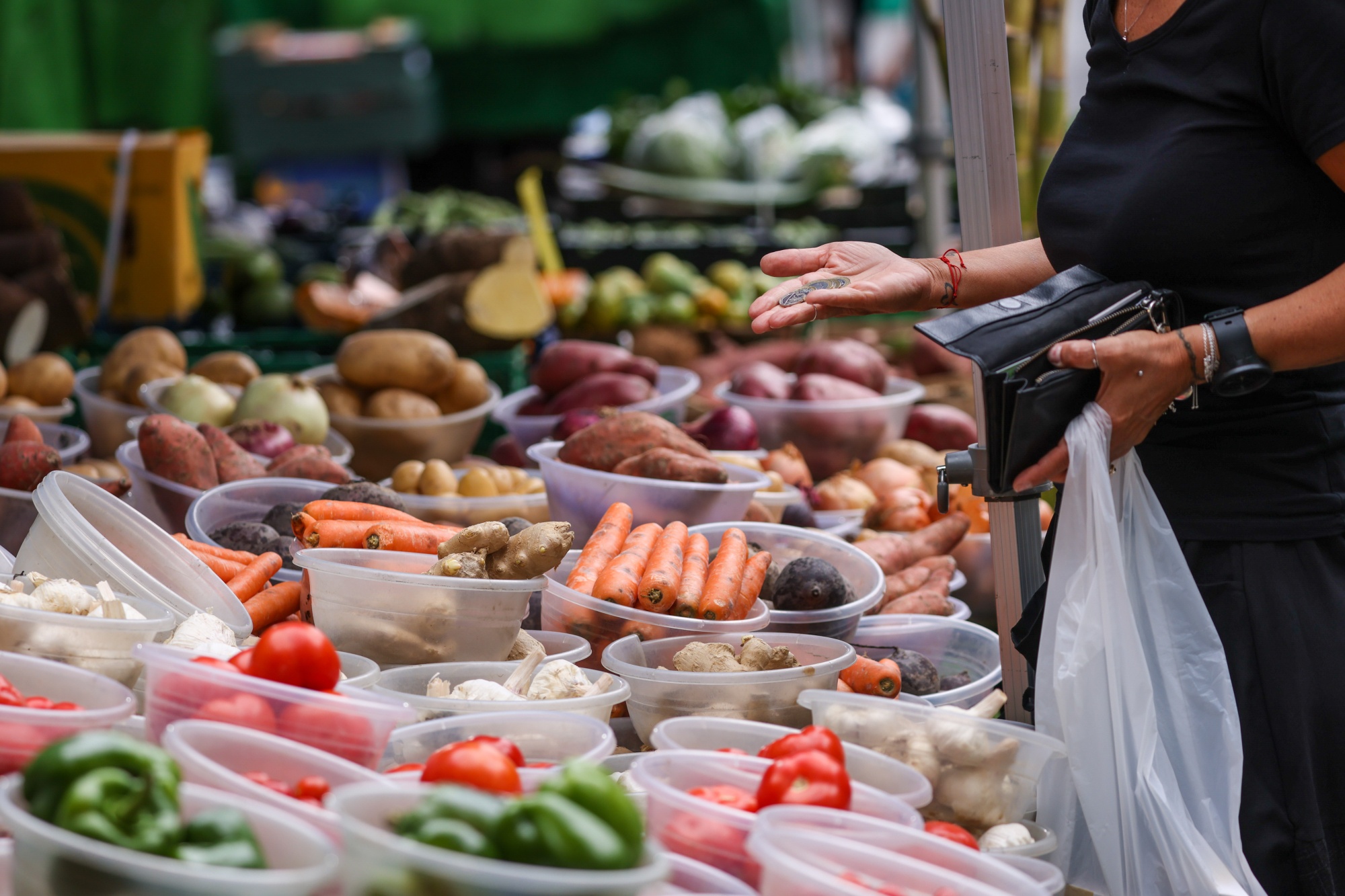In this vibrant farmer's market scene, you are surrounded by a plethora of fresh produce meticulously arranged in small, clear plastic bowls. The foreground is dominated by an array of vegetables including green peppers, red and medium-sized tomatoes, garlic, carrots, onions, and potatoes, both brown and red. Sweet potatoes are also visible among the neatly organized bowls. In the right-hand side of the image, a woman dressed in all black with a black watch and red bracelet holds a white grocery bag in her left hand, while her right hand is outstretched, offering change as if to pay a shopkeeper. She clutches a black wallet in her left hand, and a silver ring adorns her thumb. The background shows more containers of mestilos and possibly cabbage or lettuce, albeit slightly out of focus, enhancing the bustling and lively atmosphere of the market.